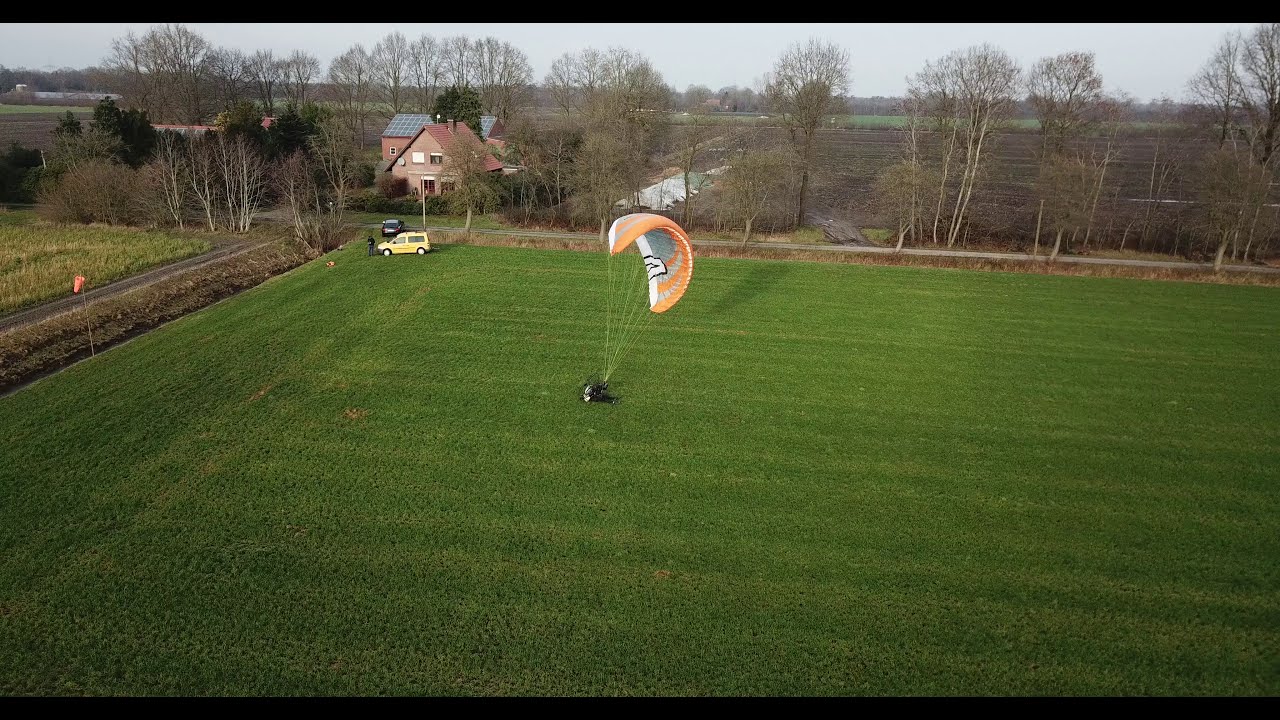This color photograph, captured by a drone, depicts a realistic and detailed aerial view of a landscape in winter. Dominating the image is a large, rectangular grassy field that occupies most of the frame. At the center of this field, a paraglider has just landed, with their yellow, orange, and blue parachute still deployed overhead. The person appears to be seated on the ground, surrounded by strings connecting them to the parachute. 

In the upper portion of the image, slightly to the left, stands a beige two-story house. In front of this house, a yellow van and a black car are parked, with a man standing next to the van. Nearby, a small road runs parallel to the field. The background reveals a landscape of multiple dead trees, evergreens, and additional grassy areas, indicating a typical winter scene. The sky above is depicted in shades of gray, emphasizing the overcast conditions of the day. No text is present in the image, allowing the viewer's attention to focus on the detailed and realistic depiction of the serene outdoor setting.